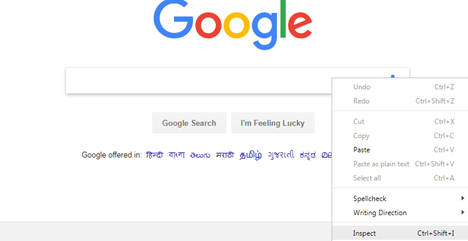The image is a screenshot of a Google search page with a clean, white background. Prominently featured at the top center is the iconic Google logo, composed of a capital 'G' in blue, followed by a lowercase 'o' in red, another lowercase 'o' in yellow, a lowercase 'g' in blue, a lowercase 'l' in green, and finally a lowercase 'e' in red. Beneath the logo is a rectangular search field, inviting users to type in their queries. Directly below the search field are two gray buttons: the first one labeled "Google Search" and the second one labeled "I'm Feeling Lucky."

Below these buttons, the text "Google offered in" appears in a darker gray, followed by a list of non-English language options written in purple characters, suggesting Google’s availability in multiple languages.

To the right side of the screen, partially overlapping the search field, is a drop-down menu panel. This menu displays several options in gray text, outlining various browser actions with corresponding keyboard shortcuts:

1. **Undo** - **Control + Z**
2. **Redo** - **Control + Shift + Z**
3. **Cut** - **Control + X**
4. **Copy** - **Control + C**
5. **Paste** (bold) - **Control + V**
6. **Paste as plain text** - **Control + Shift + V**
7. **Select all** - **Control + A**

Further down the menu, in darker type, it says **Spell Check** followed by a right-facing caret (►), indicating more options. Below this, it says **Writing Direction** with another right-facing caret (►).

At the bottom of this menu, a gray band features the option **Inspect**, labeled with the shortcut **Control + Shift + I**.

This detailed description captures the essence of a typical interaction with the Google search engine, providing a clear image of the visual and interactive elements on the screen.